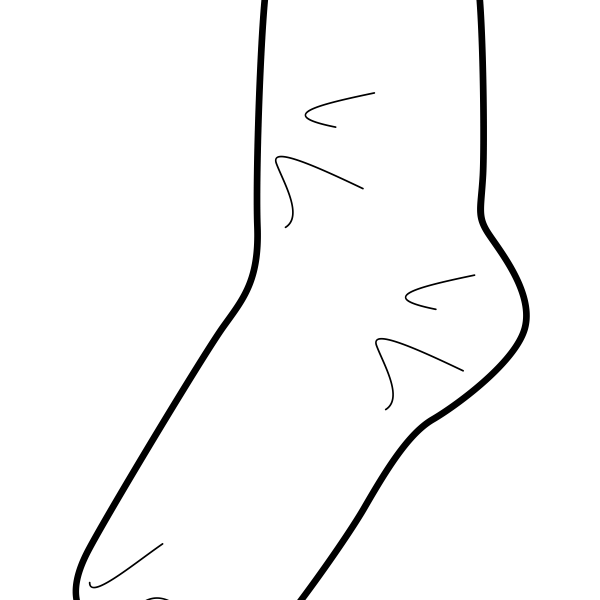The image is a black and white outline of a shape that appears to resemble a part of a foot. The sketch features a thick black outline with minimal detail, primarily drawn in a side view. The top part of the outline curves inwards and then outwards at an angle on both sides, which could represent an ankle or heel. The bottom of the outline is cut off where the toe area would typically be. Inside the outline, there are a few squiggly lines, five to be precise, which look like hooks or possibly hair. The background of the image is entirely white, with no text or additional context to clarify the subject. The overall drawing is simplistic, only highlighting the form with black lines and leaving the rest blank.